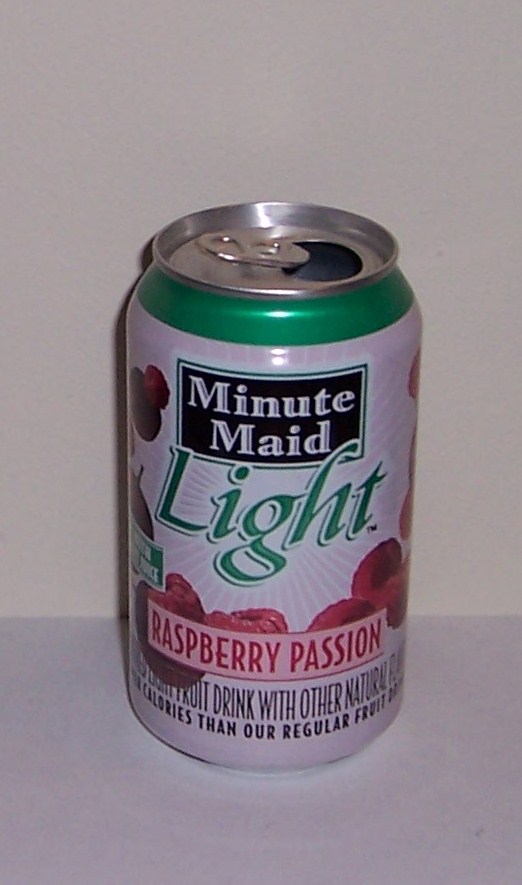This photograph showcases a Minute Maid Light Raspberry Passion drink can against a stark white background. The can itself features a distinctive design: an emerald green stripe encircles the top, transitioning to a predominantly white body that serves as the backdrop for various design elements. The prominent Minute Maid logo is displayed within a black rectangle, with "Minute Maid" in bold white letters and "Light" in striking green just below. The flavor, Raspberry Passion, is highlighted within a pink rectangle with red letters, accentuated by vivid, photo-realistic imagery of red raspberries adorning the can. The top of the can, made of silver aluminum, includes an opened pop-top. Additional text, partially obscured, mentions juice and other natural flavors at the bottom, enclosed by a thin green border. The can is set upon a gray platform that subtly blends into the background, enhancing the visual focus on the beverage.